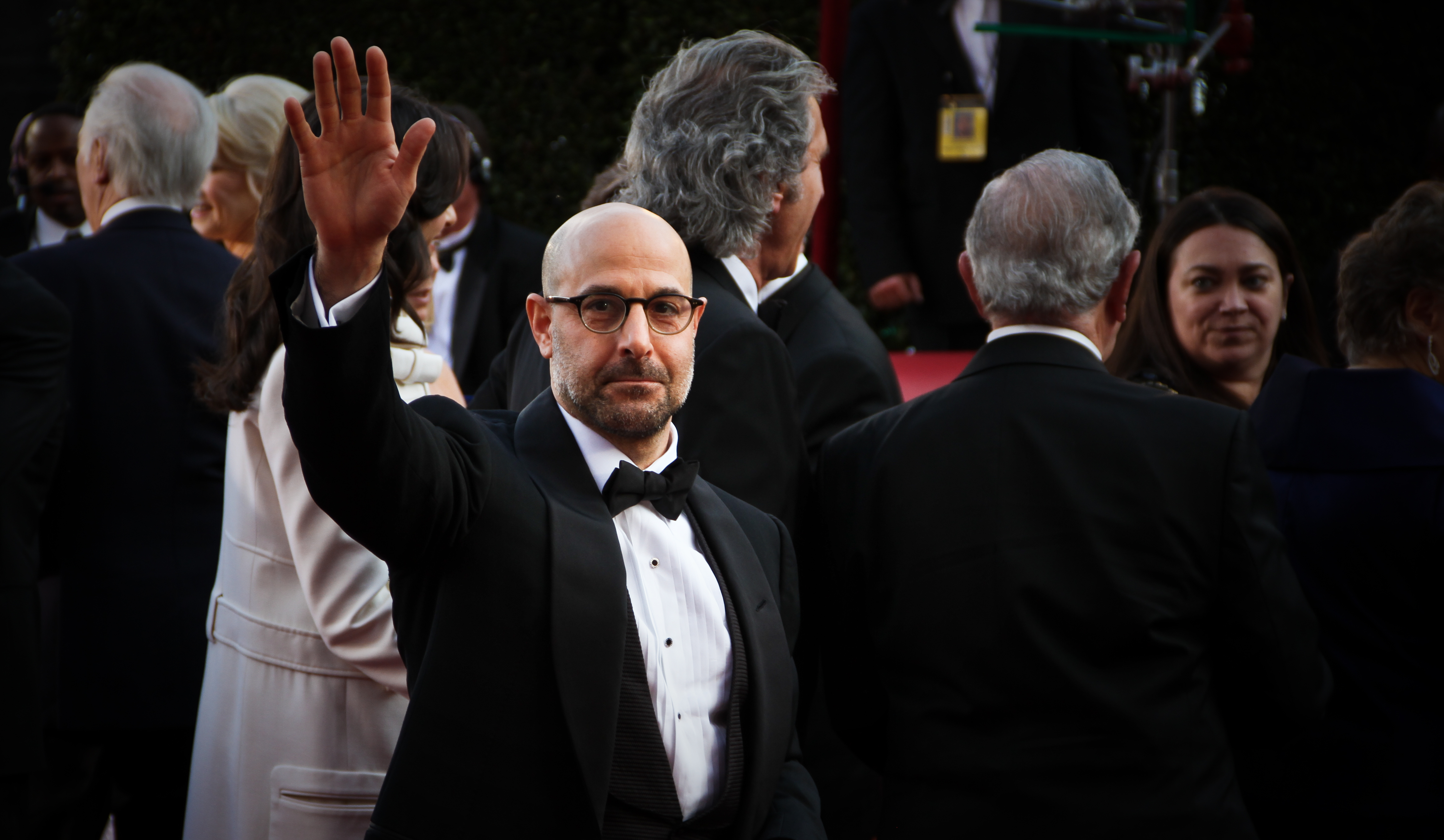In the forefront of the photograph stands a bald man with a closely trimmed black stubble beard and mustache, wearing black-rimmed round glasses. He sports an elegant black dress jacket, a crisp white dress shirt with black buttons, and a black bow tie. With his right hand raised in a friendly wave, he is the only one directly looking at the camera. Behind him, a backdrop of what appears to be a red stage lends a sense of formality to the scene, suggesting an award show or premiere event.

To the left of the man, a woman with long black hair, dressed in a light tan jacket with side pockets, gazes in the opposite direction. Other individuals surrounding them are also dressed in formal attire, with several men and women visible, most seen from the back. The overall composition and attire of the people suggest a gathering of celebrities or high-profile figures, underscoring the importance of the man leading the photograph.